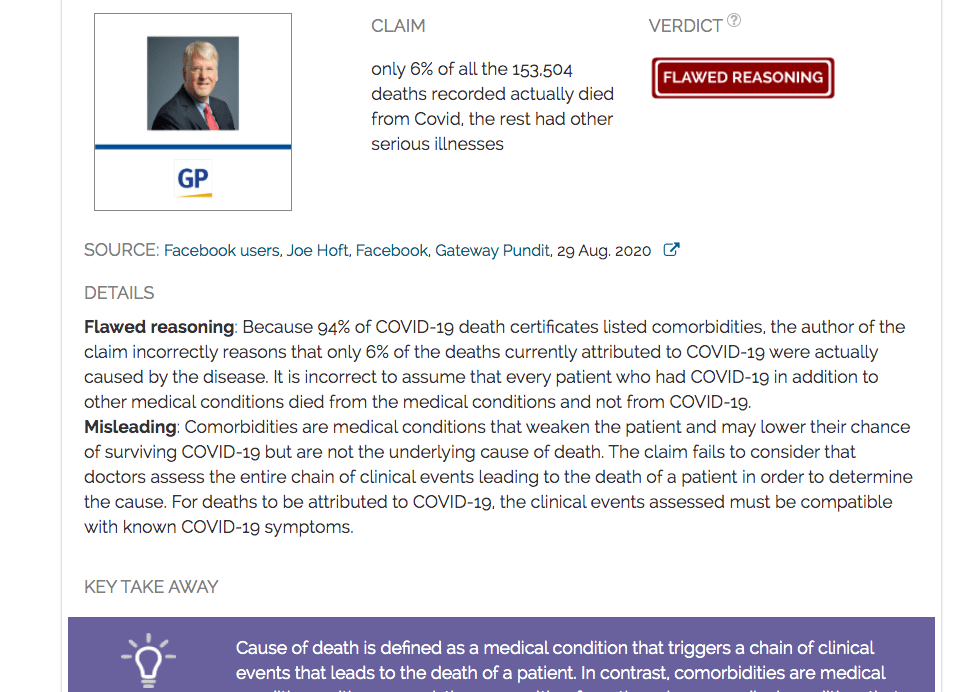The webpage in the image appears to be a segment from a fact-checking website. It features a profile picture of an older white man with gray hair, positioned on the left side of the page. Beneath his image is a logo labeled "GP." To the right of the photo, there is a section titled "Claim," which discusses the number of deaths attributed to COVID-19 versus other illnesses.

A "Verdict" section is prominently featured with a large red-bordered button that reads "Flawed Reasoning." Below this segment, various paragraphs provide additional context, including sections labeled "Source," which offers links to different references, and "Details," which explains why the reasoning is considered flawed and provides supporting arguments.

Further down, there is a section titled "Key Takeaway," although the content cuts off at this point. At the bottom of the page, within a blue-bordered box featuring a light bulb icon, a note explains that the cause of death is defined by the primary medical condition that initiates the sequence of clinical events leading to the patient's death, as opposed to comorbidities. The page cuts off again, leaving the description incomplete.